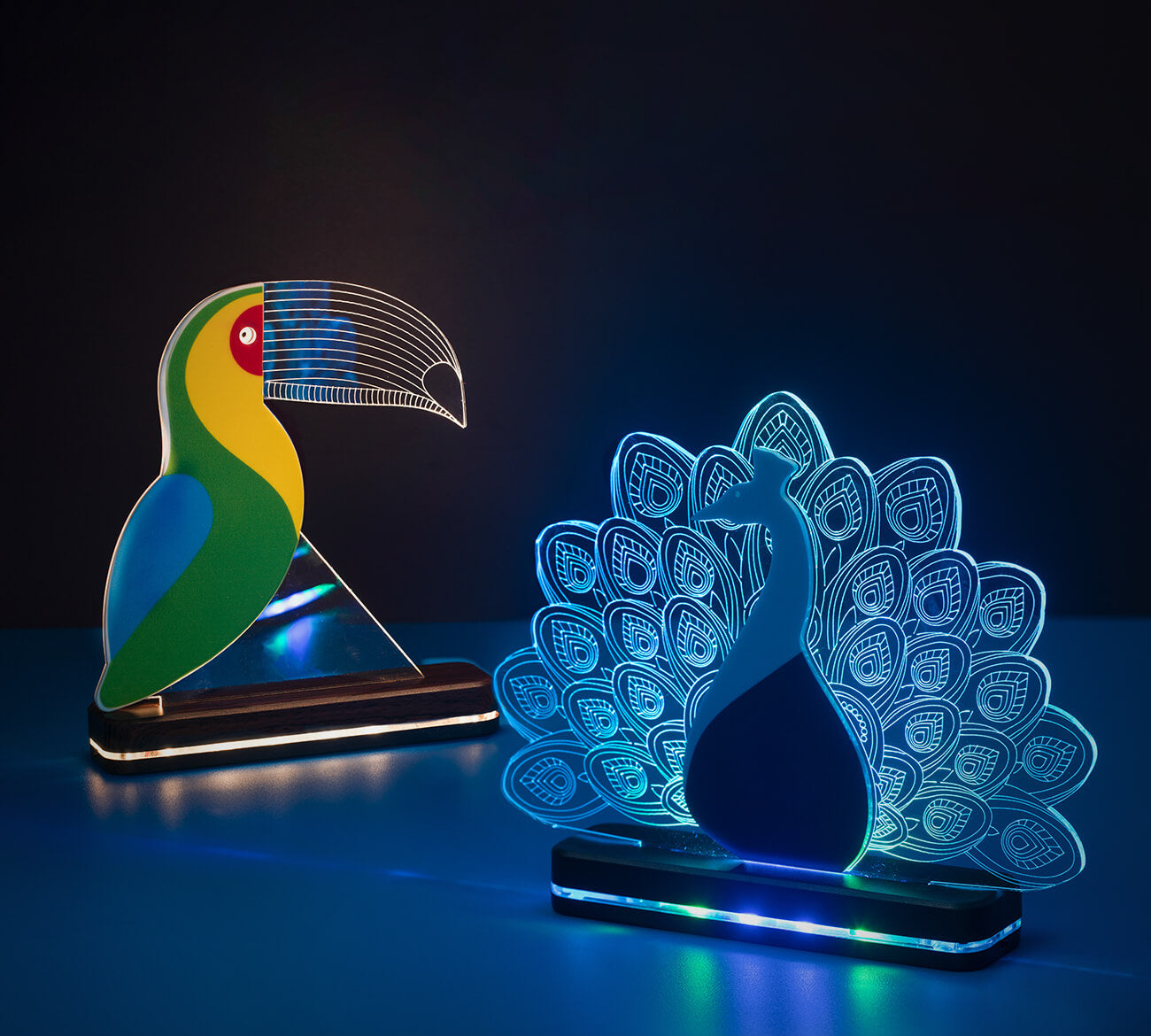This photograph captures two vibrant and contemporary neon art pieces, both depicting birds. On the left is a multicolored toucan, adorned with segments of green, yellow, blue, and red, with a strikingly large black beak accentuated by horizontal white neon lines. The toucan's eye is highlighted in a vivid red, and its intricate design sits on a dark wooden oblong base embellished with a silver strip either emitting or reflecting light. To the right, positioned closer to the foreground, stands an ornate peacock rendered in various shades of luminous blue. The peacock's feathers are intricately detailed, showcasing a delicate pattern, and its neck and head extend upward in a lighter shade of blue. This figure also rests on a similar dark wooden base with a light-emitting silver line. Both sculptures are set against a black background on a bluish table, creating a modern aesthetic with their illuminated detailing and contemporary craftsmanship.